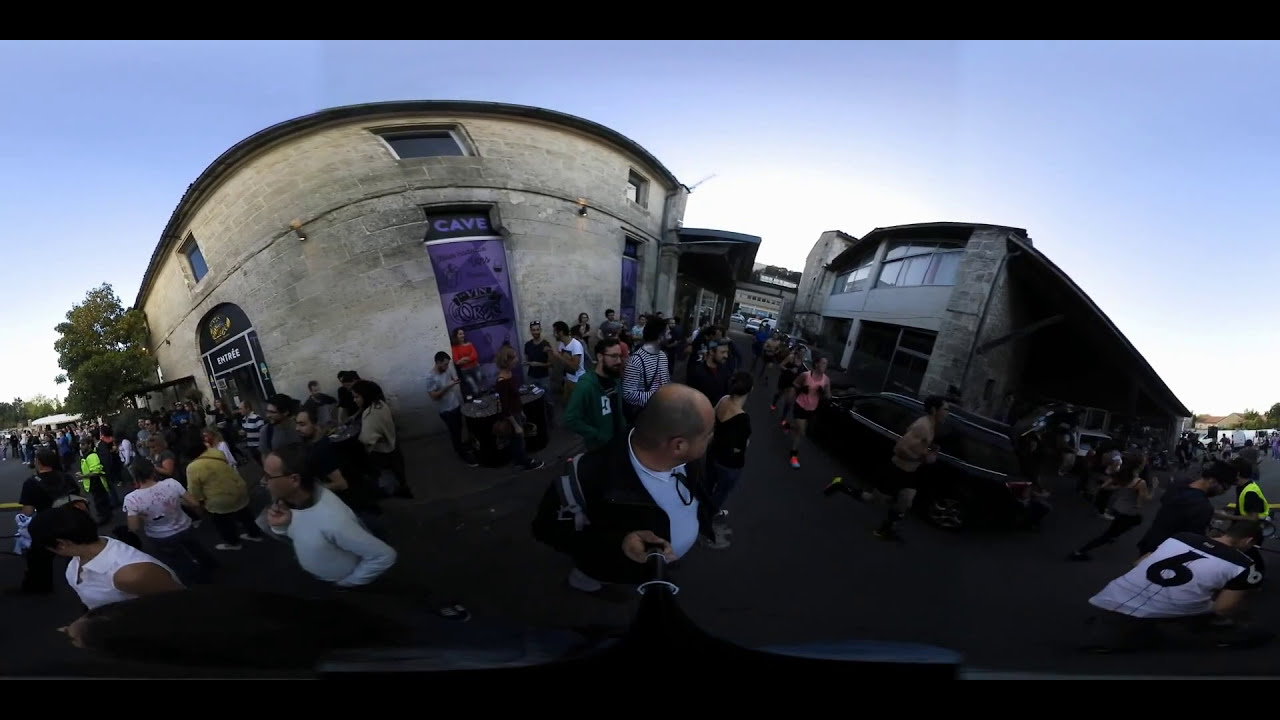The image depicts a bustling outdoor scene captured with a fisheye or 360-degree lens, creating a concave, circular effect. At the center of the photograph, a large crowd of people are walking and milling around on an asphalt road, suggesting a lively atmosphere perhaps related to a race or tourist attraction. The people exhibit a diverse range of attire: one man in the forefront wears a jacket and t-shirt, while nearby, a girl in a long-sleeved shirt and another in a sleeveless shirt can be seen. Additionally, several individuals on the right appear to be in running gear, possibly participants in a race, with other onlookers acting as spectators. The backdrop features beige stone buildings, one notably labeled with the word "CAVE" across its top. To the left, a tree adds a touch of greenery to the urban scene. At the very bottom right, a white sign with the number six is visible. The sky overhead is a light blue with some white clouds, further indicating it’s a bright day. The image’s warped effect distorts both the people and the architecture slightly, adding to the dynamic feel of the setting.